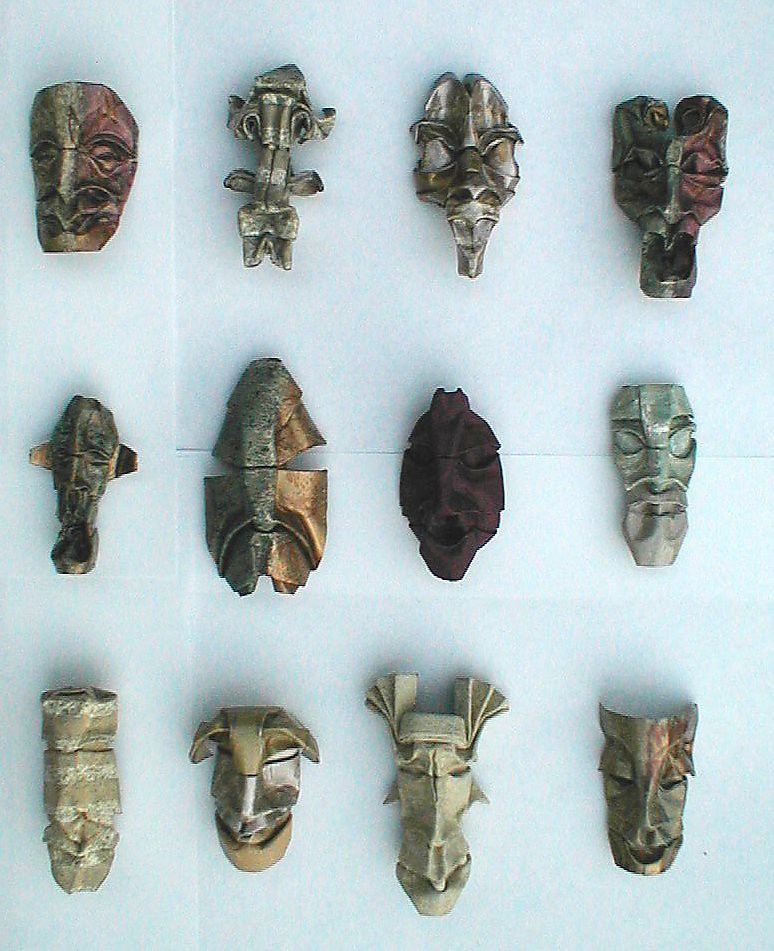This photograph showcases an array of intricate masks displayed against a light blue wall, meticulously arranged in a grid format with three rows and four columns. The masks vary significantly in design and material, some exuding a metallic sheen with colors ranging from bronze and reddish hues to gray and silver. A distinctive bronze mask features a reddish side and a grayish side, resembling a face, while another silver one has an elongated snout. Among the collection, there is also a mask resembling a tiny man, and another large one that appears to cover the entire face. One mask at the bottom strikingly resembles a drum with a face painted on it. The masks, varying in tribal, stone-like, and painted brown designs, display a myriad of features such as wide mouths, closed eyes, angular noses, and sharp cheekbones with inward-turning horns. Some exhibit animal-like characteristics, with long faces and side-positioned ears.